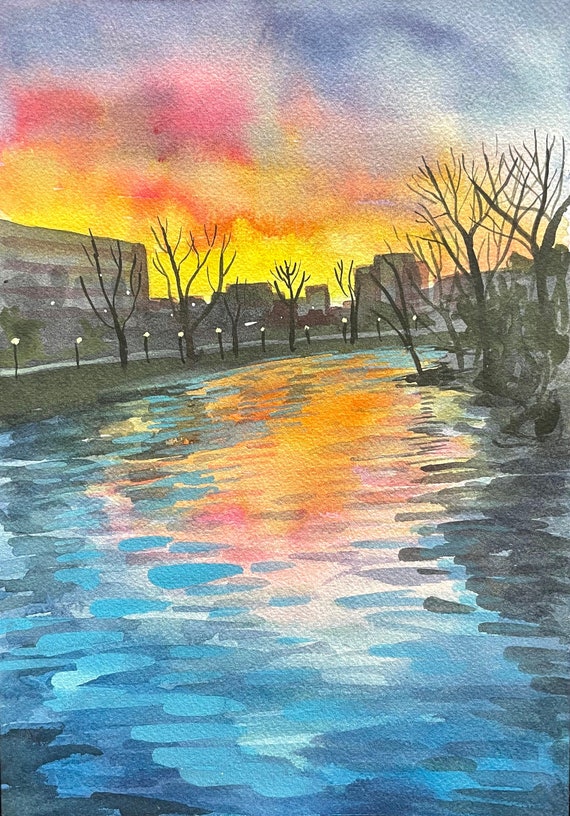This painting, likely created with a combination of acrylic and watercolor techniques, presents a serene riverscape at sunset. The expansive river, spanning more than half of the composition, reflects the vivid colors of the sky, which transitions from deep purples and blues at the top to warm yellows and reds at the horizon. On either side of the river, leafless trees, painted in stark black, create a silhouette against the glowing sky. The banks of the river feature light poles that add a subtle golden hue to the scene. In the background, a cityscape emerges with buildings rendered in shades of brown, black, grey, and accented with red and white lines, providing a harmonious contrast to the natural elements. The city lights add a touch of warmth, suggesting the onset of evening. The overall effect is a contemplative, picturesque moment captured in vibrant, reflective water and a colorful sky.